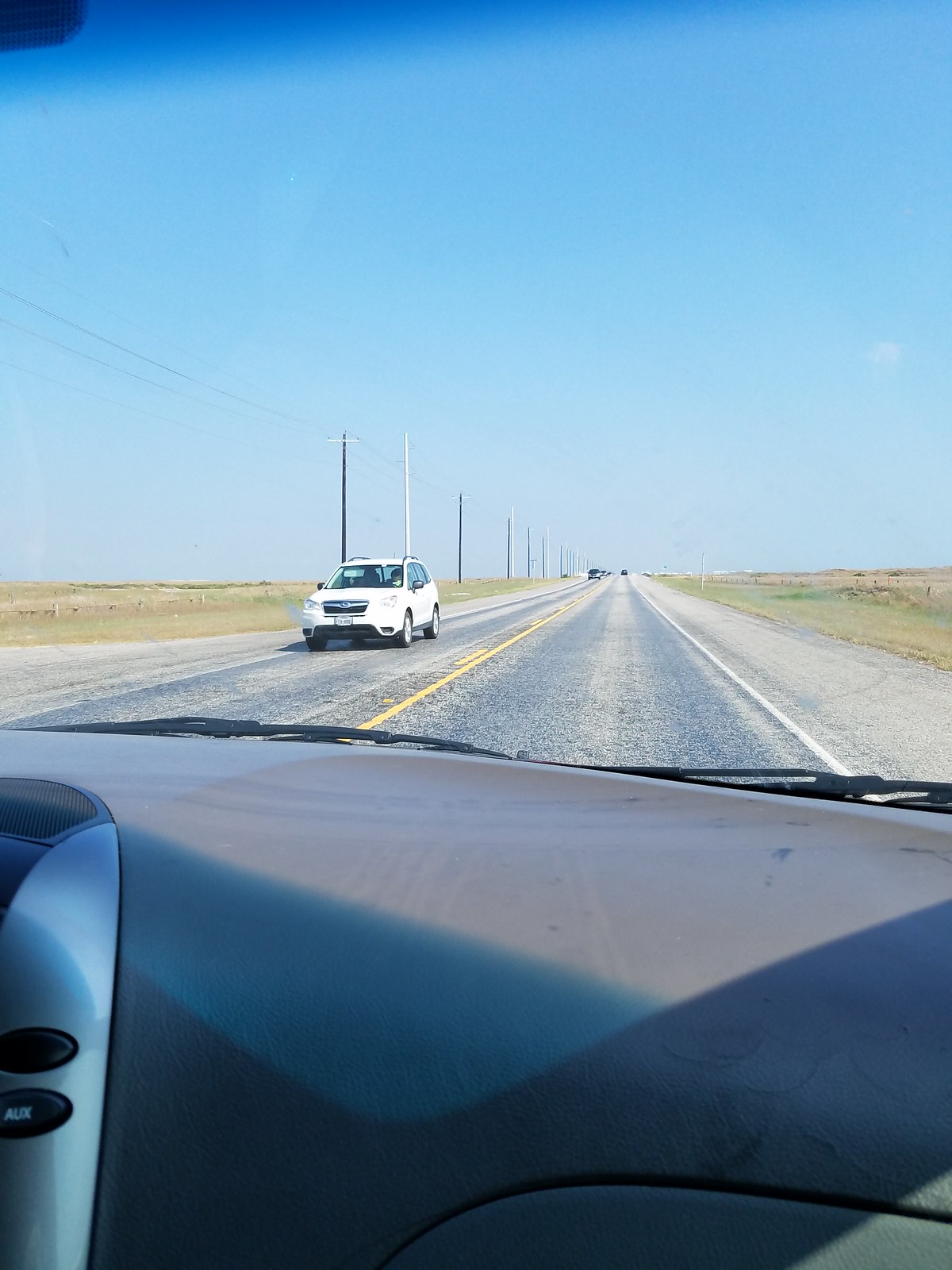The photograph, taken from the passenger seat of a vehicle, captures a scenic two-lane, one-way road extending into a rural area under a clear blue sky. The dashboard of the car, which has a gray hue and features a center control panel with two oval-shaped black buttons on a silver panel (one marked with 'AUX'), occupies a significant part of the foreground. Visible on the dashboard is a speaker grill on the left side and the windshield wipers positioned centrally.

The road itself, composed of a concrete and asphalt mix, is marked with white lines on either edge and a combination of yellow and white lines down the center. To the left side of the road, there are pylons and power lines running parallel to the road, while on both sides, fields of short grass and fences demarcate the rural landscape. A white car is visible in the oncoming lane, with other vehicles further down the road. The sky above is mostly clear, with a single white cloud in the top right corner, framing the picturesque drive through this tranquil countryside.